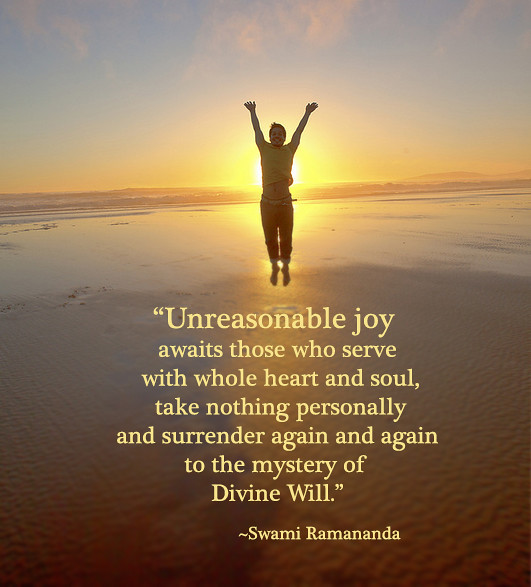The image features a computer-generated sunset or sunrise scene at a tropical beach, where a man, likely with brown hair, is joyfully leaping into the air, his feet off the ground and arms stretched upwards. He wears a t-shirt revealing his midriff and long pants. The backdrop includes the vibrant, setting sun casting an orange hue over the clear waters and sandy shore. In light yellow text, a profound quote by Swami Ramananda overlays the scene, reading: “Unreasonable joy awaits those who serve with whole heart and soul, taking nothing personally and surrendering again and again to the mystery of divine will.” The text is presented in quotation marks with the author's name beneath.